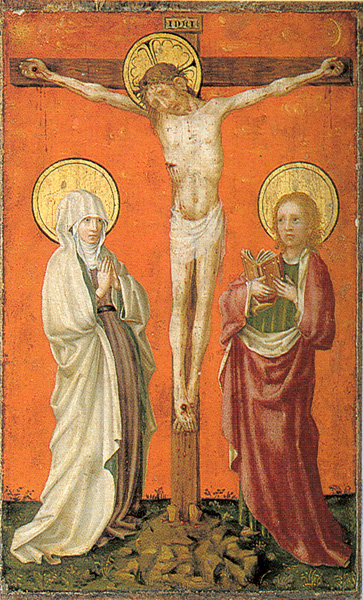In this detailed Byzantine medieval painting, a scene of the crucifixion is depicted with striking contrast between the three-dimensional, realistic faces of the figures and the otherwise two-dimensional background. At the center, Jesus hangs emaciated on a wooden cross, his thin, pale body showing wounds with blood dripping from the spikes through his hands and feet and a slit under his ribs on the left side. A golden halo with intricate black designs floats above his head, and an inscription reading "INRI" is posted at the top of the cross, though some details are faint.

On either side of Jesus stand two women, both adorned with golden halos. On the left, a woman in a white robe that drapes to the ground and covers her head stands with her hands clasped in prayer. She has light skin and is believed to represent Mary, the mother of Jesus. On the right, a woman with auburn hair and fair skin holds an open book close to her chest, dressed in a red robe over a green suit. This woman, thought to be Mary Magdalene, appears deeply concerned. 

The background is a solid orange hue, and the foreground depicts a rocky, brown soil with hints of green. This intricate artwork blends elements of depth in the faces and attire of the figures with a pronounced flatness in the overall composition, emphasizing the emotional poignance of the crucifixion scene.